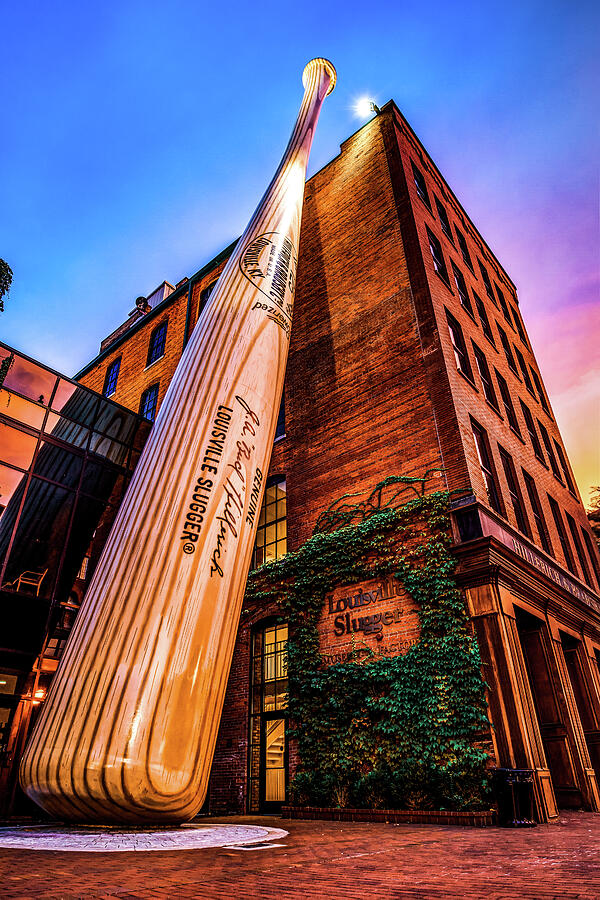This detailed photograph captures the imposing and captivating facade of the Louisville Slugger building, depicted in a rich, dark brown brick extending six to seven stories high. A defining feature of the image is the colossal Louisville Slugger baseball bat, which towers above the roofline, leaning majestically against the side of the building. This bat, bearing the iconic Louisville Slugger name, draws the viewer's eye immediately. The building's exterior is further adorned with ivy crawling up the brick walls, adding a touch of nature to the urban scene. A plaque bearing the Louisville Slugger name is nestled among the greenery, subtly integrating branding into the natural decor. The sky above transitions from vibrant blue to a blend of soft pinks, yellows, and whites, adding a dynamic and picturesque backdrop. Additionally, the entire structure sits on a brick walkway that encircles the building. Elements such as entrances with brown wooden panels and potentially a small figure or light stand out at the roof's edge, completing this visually rich and storied composition.